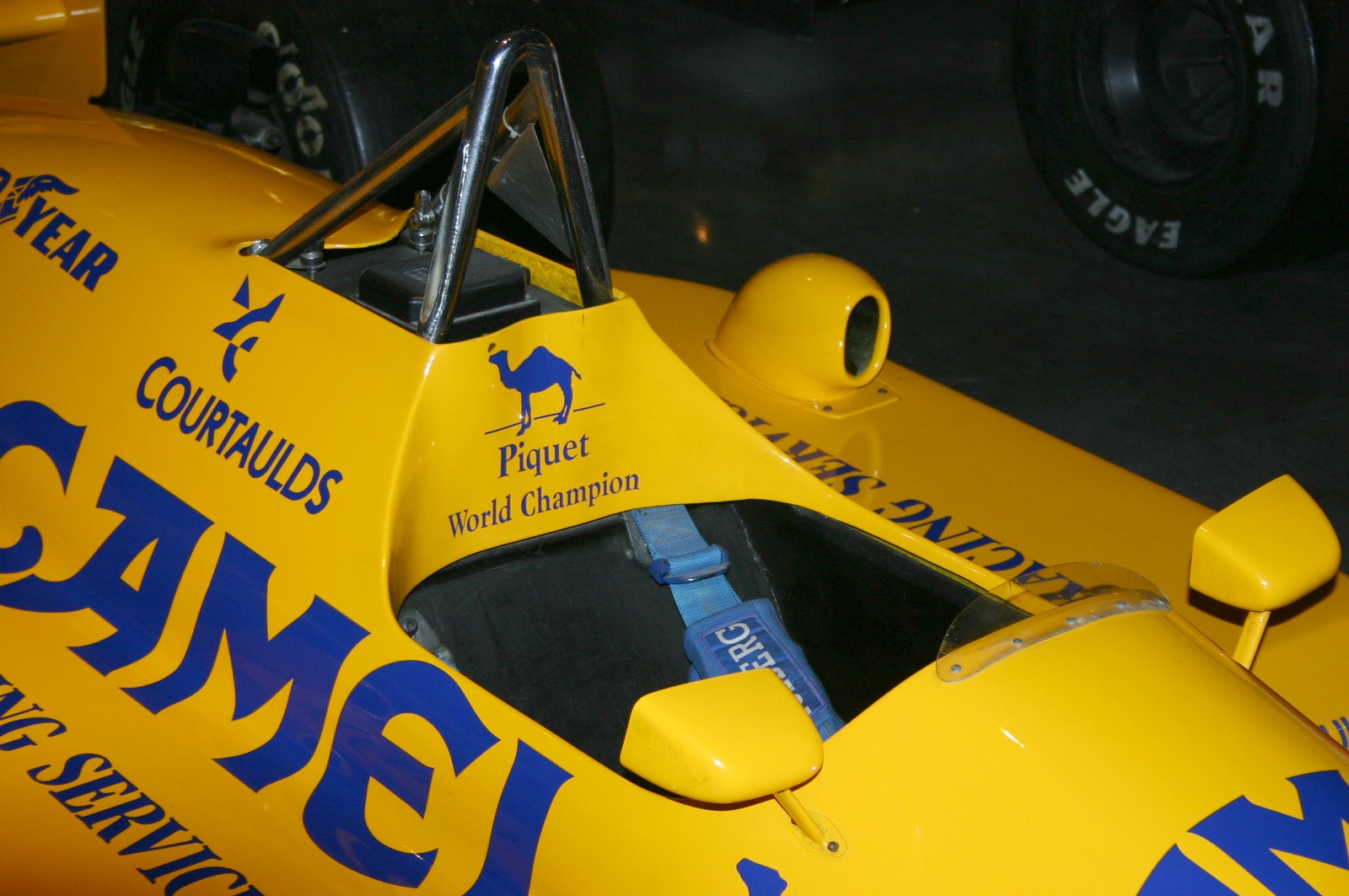The image features a predominantly yellow race car with a sleek, molded one-seater cockpit area. The seat is black with a padded blue seatbelt that has the letters "ERG" visible in white text. Behind the seat, "Piquet World Champion" is inscribed, accompanied by an illustration of a camel. On the left side of the vehicle, the sponsor "Courtaulds" is displayed, followed by the larger text "camel" and a partially visible word ending in "G" under the term "service." The rear view mirrors on each side of the cockpit and a small exhaust fan towards the back right are noteworthy details, along with a blue symbol resembling a yellow square bisected by a blue line and a curved half C below. The car is equipped with Goodyear tires, labeled as "Eagle" on the upper right, consistent with its road racing design. Above the seat area, additional sponsors such as "Goodyear" are visible, enhancing the car's highly sponsored appearance. The vehicle is positioned on a dark asphalt surface.